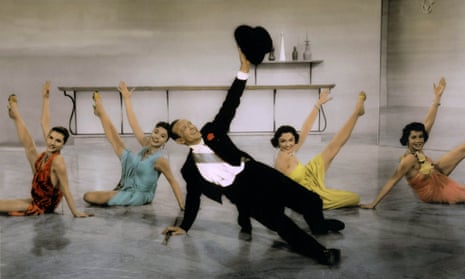In a scene likely from a classic movie, possibly featuring the iconic Fred Astaire or Frank Sinatra, a man dressed in a black tuxedo with a white shirt and a red boutonniere is performing a dance move on the ground. He is elegantly posed with one arm supporting him on the floor and the other holding a black top hat aloft. His legs are splayed out in front of him in a graceful stride. Surrounding him are four female dancers, positioned in a line behind him, mirroring his pose with one hand on the ground and the other arm and leg raised. Each woman is dressed in a vividly colored dress: red, light blue, canary yellow, and coral pink. They all have dark hair and are seated on a concrete floor with a gray wall behind them, suggesting a dance studio setting. In the background, a shelving unit adorned with four vases adds to the scene's ambiance.